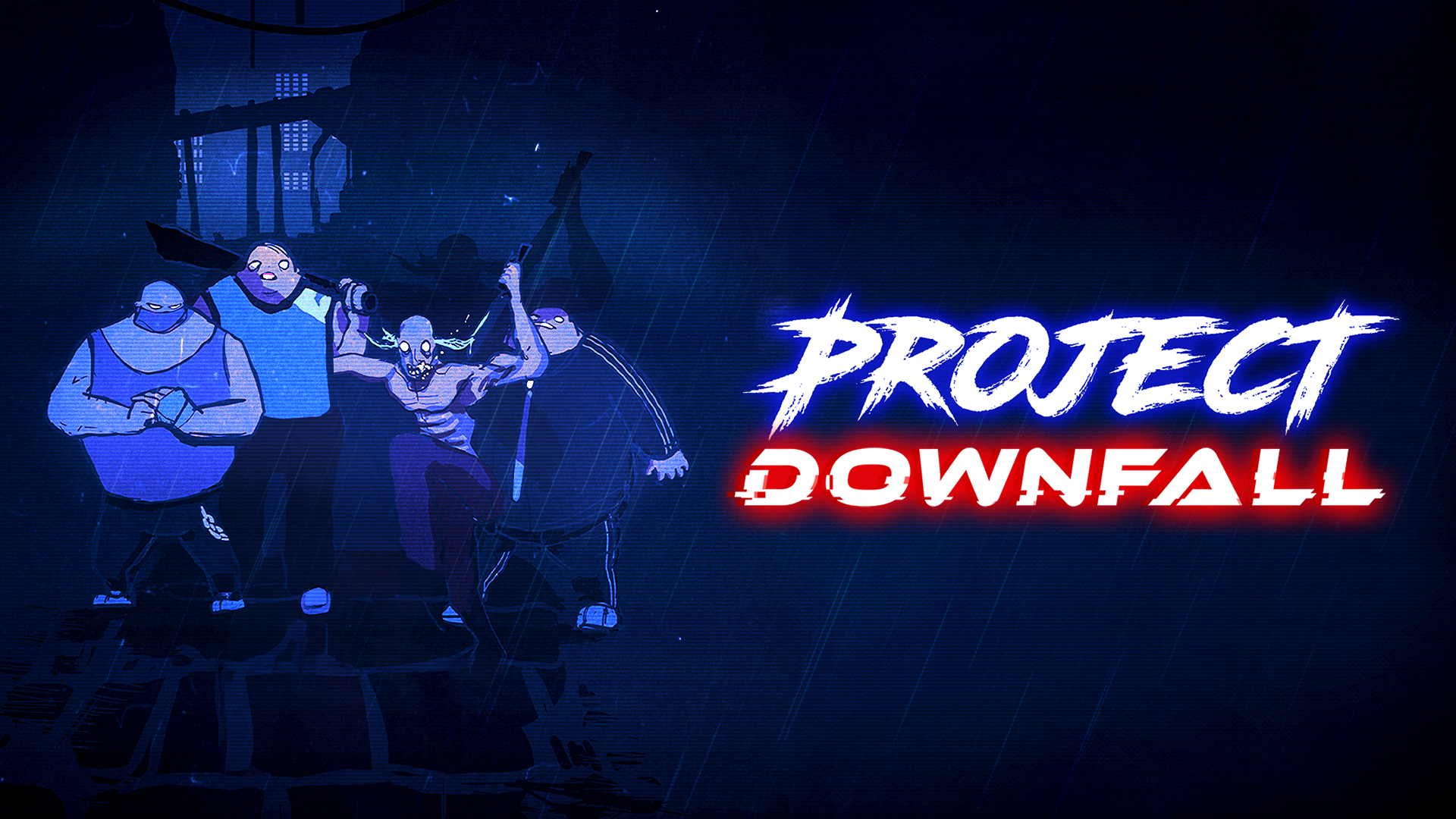The image showcases a scene reminiscent of video game art or a video thumbnail, depicting a dark, rainy alleyway at night with four distinct cartoon-like characters standing on a black stone street. On the left, a very large, fat man wearing a blue tank top, black pants, and a bandana over his mouth stands with his fists clenched. Next to him, a man in a short-sleeve white shirt and black pants holds a bat or club over his shoulder. To his right, a crazed, wide-eyed, shirtless man with a gray mask, sparse wispy hair, and purple pants brandishes a rifle. Finally, on the far right, there is another very large, fat man wearing a black Adidas tracksuit. The entire scene is shrouded in a dark, blue-hued atmosphere with visible rain streaks. 

On the right side of the image, glowing white text reads "PROJECT DOWNFALL," with "PROJECT" appearing in sketchy, all-capital letters outlined in a blue glow, and "DOWNFALL" in bold, futuristic text with a red glow. The title is centered at the top against a black and purple background, completing the dramatic and intense composition.